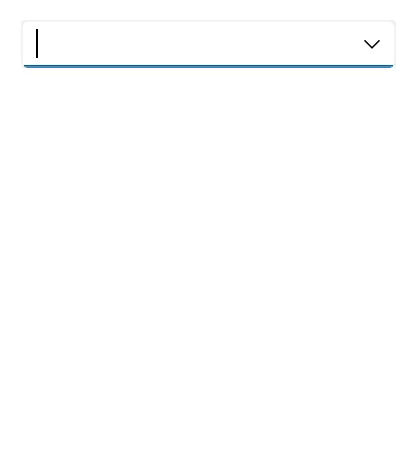This animated GIF showcases a drop-down menu featuring a variety of social media platforms. At the top of the menu, there is a search bar accompanied by a small downward-pointing arrow. In the animation, a user first types the letter "I," upon which "Instagram" is highlighted and selected. Then, the user deletes their entry and types the letter "F," selecting "Facebook" from the options. The available social media sites in the drop-down menu include Facebook, Google+, Instagram, LinkedIn, Skype, Telegram, and TeleVZR. The interface is simple, with a white background and black text, making the options easy to read. This GIF effectively illustrates the functionalities of the drop-down menu and its responsive search features.